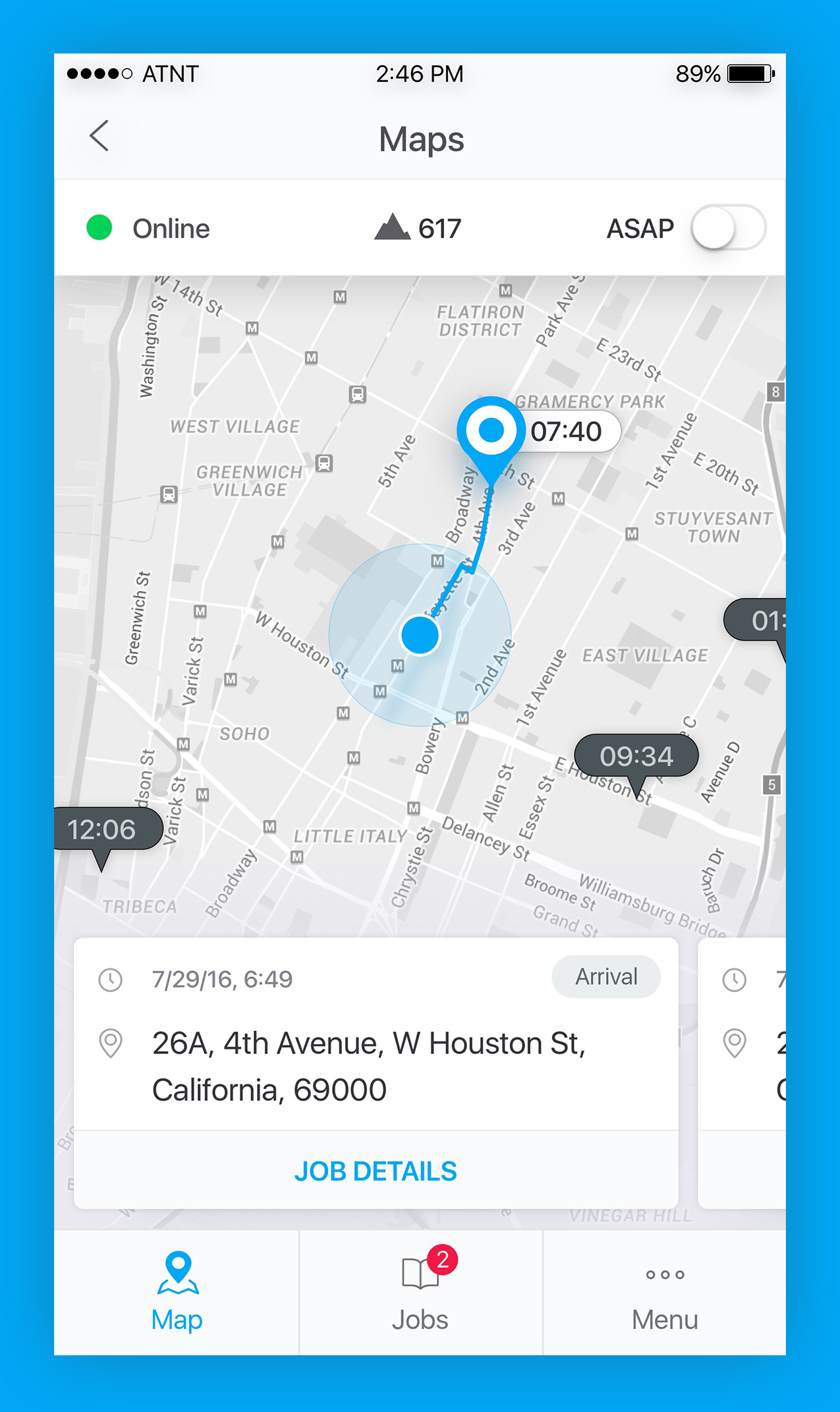A screenshot from a cell phone displaying a map interface is captured within a blue-bordered frame. The cell phone screen features a predominantly white background with a gray top banner displaying standard status indicators: four out of five filled signal dots on the top left, the text "AT&T," the time "2:46 PM" in the center, and a battery level indicator showing "89%."

Below the gray banner, the main header is labeled "Maps" with a back arrow on the left. A white section underneath contains a green dot labeled "Online," followed by a volume or mountain symbol and the number "617." A circular slide button is labeled "ASAP."

At the center of the screen, a gray map displays various place markers and time stamps. On the bottom left of the map, the time "12:06" is visible, while "9:34" is noted on the right, with another time partially visible starting with "1" on the far right. In the center of the map, a dark blue dot is connected by a line to a blue pinhead encircled by white, with "7:40" noted nearby.

Below the map, a white square prominently displays the text "729.16.649 arrival." Further details include an address, "26A 4th Avenue, West Houston Street, California 6900." To the right of this, "job details" is written in blue next to a pin and clock icon partially showing the numbers "2" and "7."

At the bottom of the screen, icons are visible: a blue map icon labeled "Map" on the bottom left, a "Jobs" icon resembling an open book with a red notification labeled "2," and a menu with three dots on the bottom right.